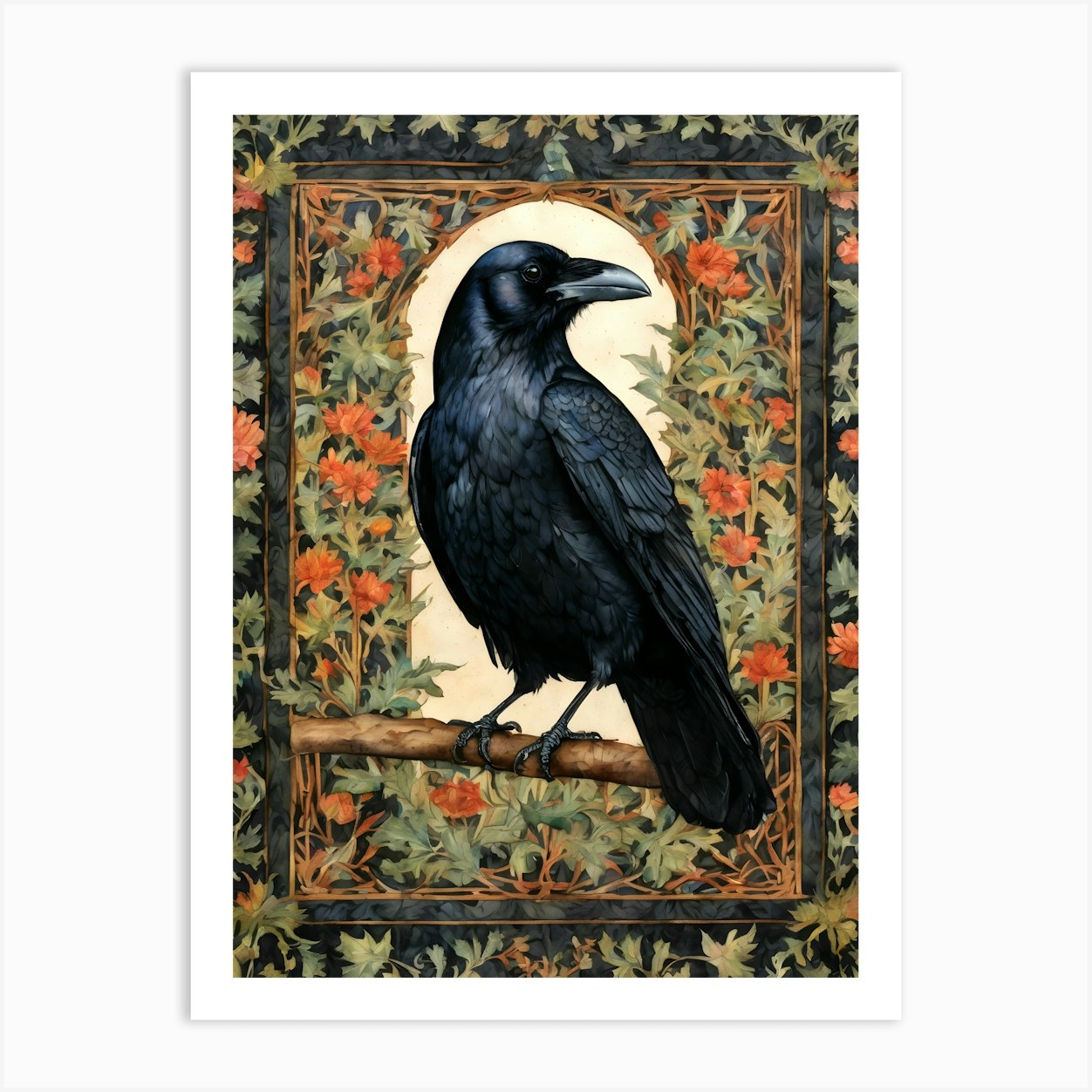The image depicts a painting of a crow-like black bird perched on a branch. The bird's body is oriented to the left, but its head is turned to the right, showcasing its long, thick gray beak which is rounded on top. Its mostly black plumage has subtle hints of light blue, purple, and grayish hues, with a slight white reflection in its otherwise dark eye. The bird's claws grip the brown branch tightly. The surrounding scene features a mix of vibrant flora with green leaves, and flowers in shades of orange, red, and yellow. Immediately behind the bird is an open arched space framed by a blue-lined square, beyond which lies another section adorned with pale green and orange plants, all encapsulated by a white border. The overall composition hints at the bird perched in front of a painted frame and window, evoking an image of nature framed artfully.